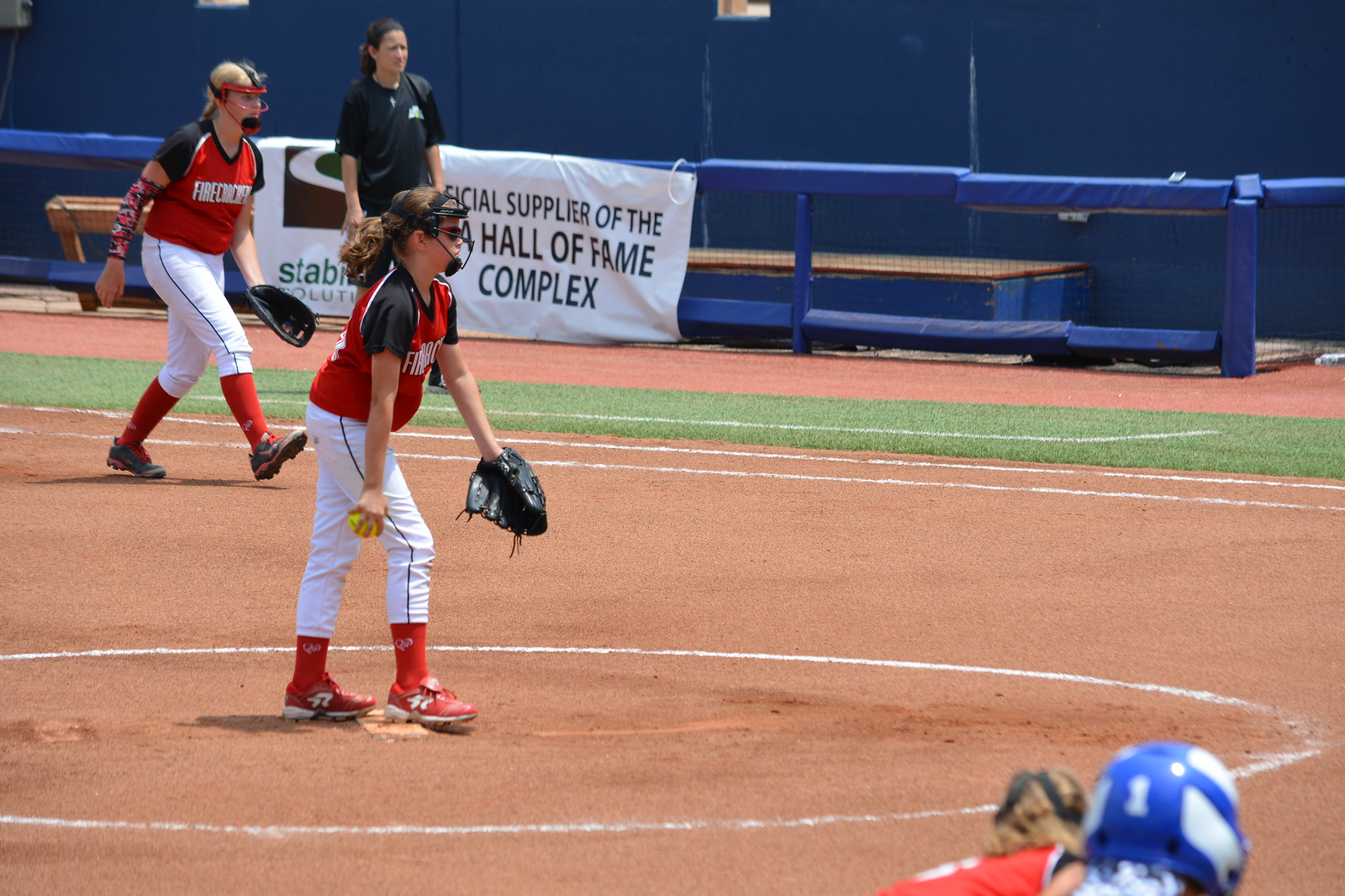The photograph captures a girls' softball game, specifically focusing on the pitcher's mound and some of the surrounding area. At the center, the pitcher stands poised with a neon yellow softball in her hand. She wears a red jersey with black sleeves, white pants with a thin stripe down the side, red socks, and red shoes. Her dark hair is tied back in a ponytail, and she is equipped with a face mask and glove for protection. To her right, on the first base line, there's another player dressed similarly in a red jersey who appears to be taking a step, her blonde hair glinting in the light. A first base coach, dressed in a black shirt and with long hair, stands on the foul line, overseeing the action. The background features a blue wall and blue benches, indicating the venue is likely an outdoor field. Hanging on the fence of what looks like the dugout area, a white banner with black text reads "Official Supplier of the Hall of Fame Complex." Nearby, another player is crouched down, ready for the next play. All persons in the image are facing to the right, adding a dynamic sense of readiness to the scene.